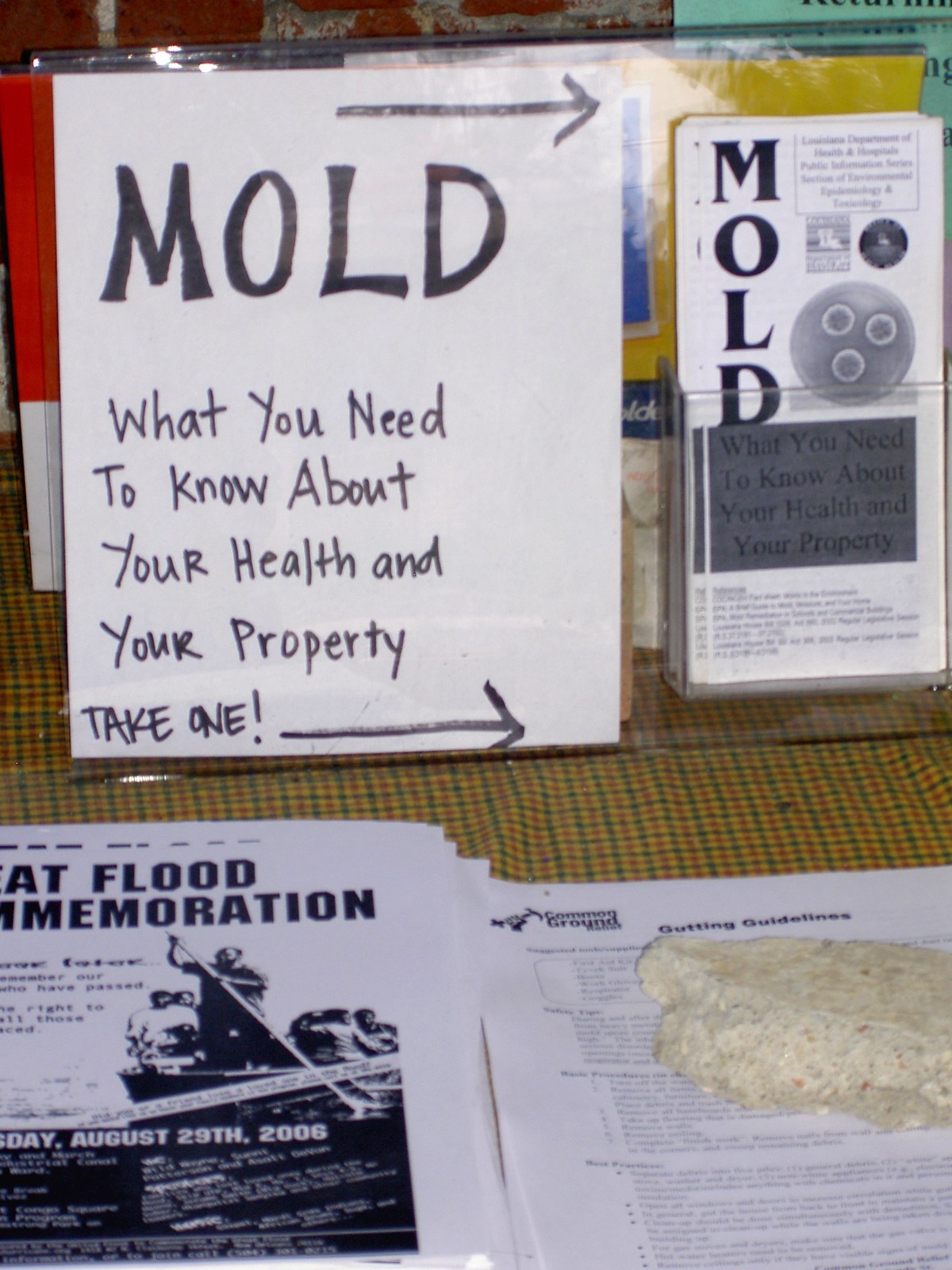This photograph captures a detailed exhibit display focused on mold awareness and its impact on health and property, likely set up on a table covered with a green, yellow, and dark orange plaid cloth. Central to the display is a paper sign that prominently reads, "MOLD: What you need to know about your health and your property. Take one." Above and below this text are arrows that draw attention to the message. 

To the right of the sign, there is a clear plastic plexiglass holder containing black-and-white brochures. These brochures echo the sign's message, with the word "MOLD" written in bold letters on the left side and a red square at the bottom, also stating, "What you need to know about your health and your property.” The front of each brochure features a photo, possibly of a mold sample in a petri dish.

In front of the brochure holder, additional handouts are scattered. One notable flyer includes an image depicting a person with a long pole in a boat, accompanied by other individuals. It reads, “AT flood MEMORATION DAY August 29, 2006." Another paper visible on the left side appears to be a white piece with bold black lettering and a black arrow pointing to the right. This document details more about the displayed topic, possibly resembling a map or other educational content annotated with small, densely packed text.